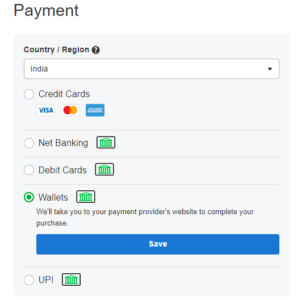The image depicts a payment screen interface. Positioned in the upper left-hand corner is the word "Payment," rendered in black, capitalized font. Directly beneath this title, a blank space separates it from a light gray box that houses the payment options.

Inside the gray box, at its top left corner, the bold, black text "Country/Region" leads the section. Adjacent to this label is an information icon, represented by a white question mark enclosed in a black circle. In the corresponding input field to the right, "India" is pre-filled as the selected country.

Continuing downward, the payment methods begin with a header labeled "Credit Cards," marked by a white bullet point. Below this header, the accepted credit card icons are displayed: Visa, MasterCard, and another blue logo which might represent a less common card. 

Further down, the "Net Banking" option is present, identified by an icon that resembles either a trash can or a bank, likely representing a banking service.

Lastly, there is an option for "Debit Cards," although no explicit details about this option are provided within the image. The currently selected payment method is "Wallets," indicating the user's preference for a digital wallet transaction.